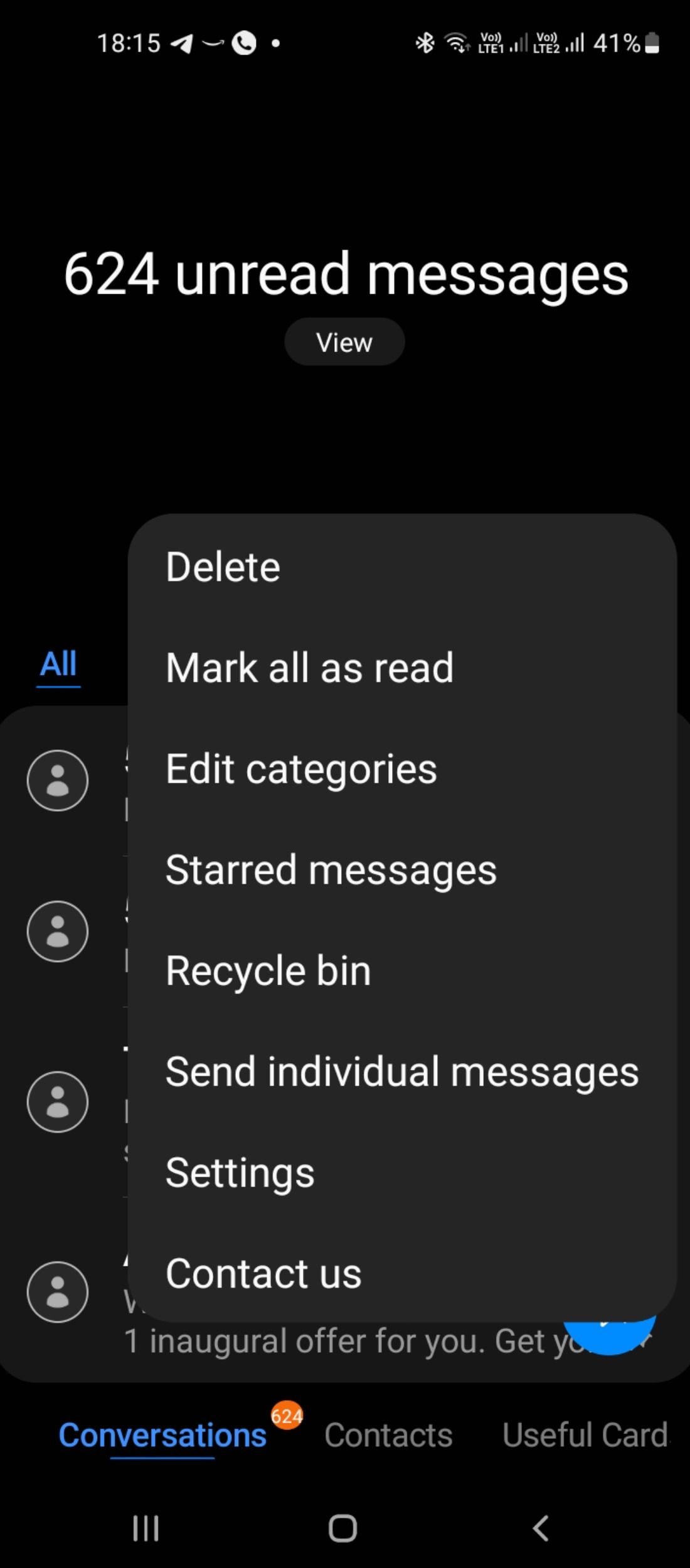The image is a screenshot from a smartphone with a black background. At the top left corner, the time is displayed in a 24-hour format as "18:15". On the top right, a battery icon indicates a charge level of 41%, along with icons for wireless connection and LTE, and a small, unreadable text that starts with the letter 'V'.

Centered on the screen, in large bold white font, is the text "624 unread messages", with the word "view" in a smaller font beneath it. Below this, there is a nearly square-shaped section with rounded corners and a dark gray background. Along the left side of this section, written in white font, but less bold, are the options: "Delete", "Mark all as read", "Edit categories", "Start messages", "Recycle bin", "Send individual messages", "Settings", and "Contact us".

At the very bottom of the screen, there is a footer with three sections. On the left, "Conversations" is written in blue. In the middle is "Contacts", and on the right side, it says "Useful card".